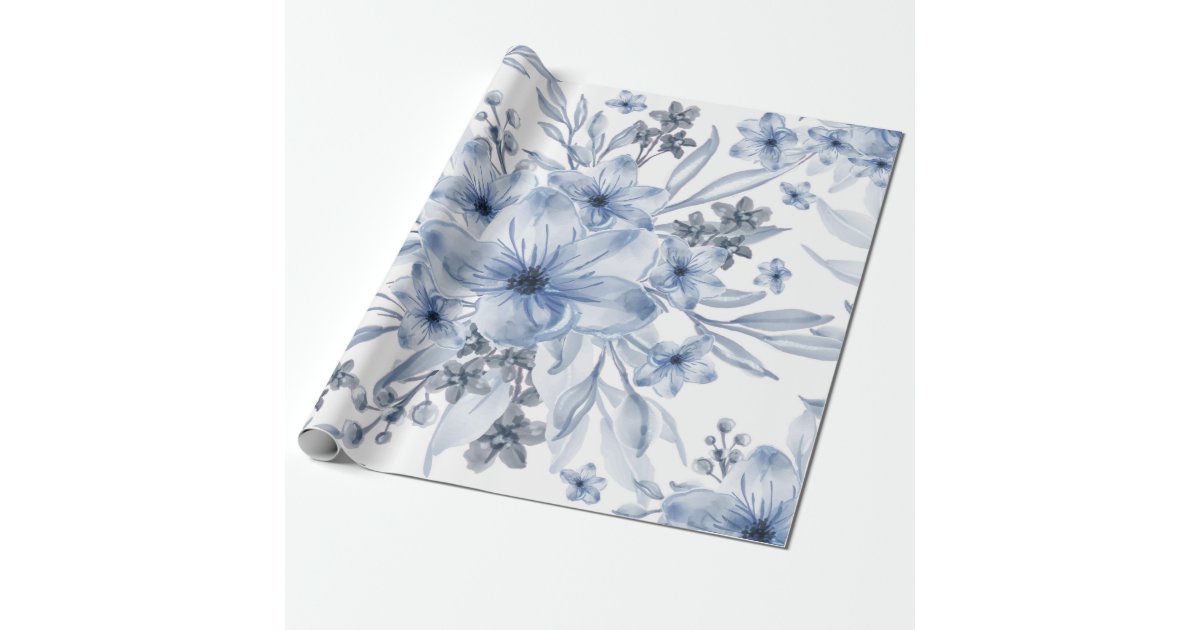This image showcases a roll of wallpaper photographed against a completely white background. The wallpaper features a white backdrop adorned with a detailed dark pen-sketch pattern. The roll, primarily situated on the left side of the image, is slightly tilted to the right at around a two o'clock position. Dominating the design are large flowers with dark centers, complemented by an array of smaller star-shaped flowers, also with dark centers. Alongside these, the wallpaper is intricately embellished with leaf stems and sporadically placed sprigs featuring twigs with berries or blossoms. The careful design work suggests a monochromatic palette, with some viewers noting a subtle blue tinge in the flowers, resembling delicate watercolor shading.